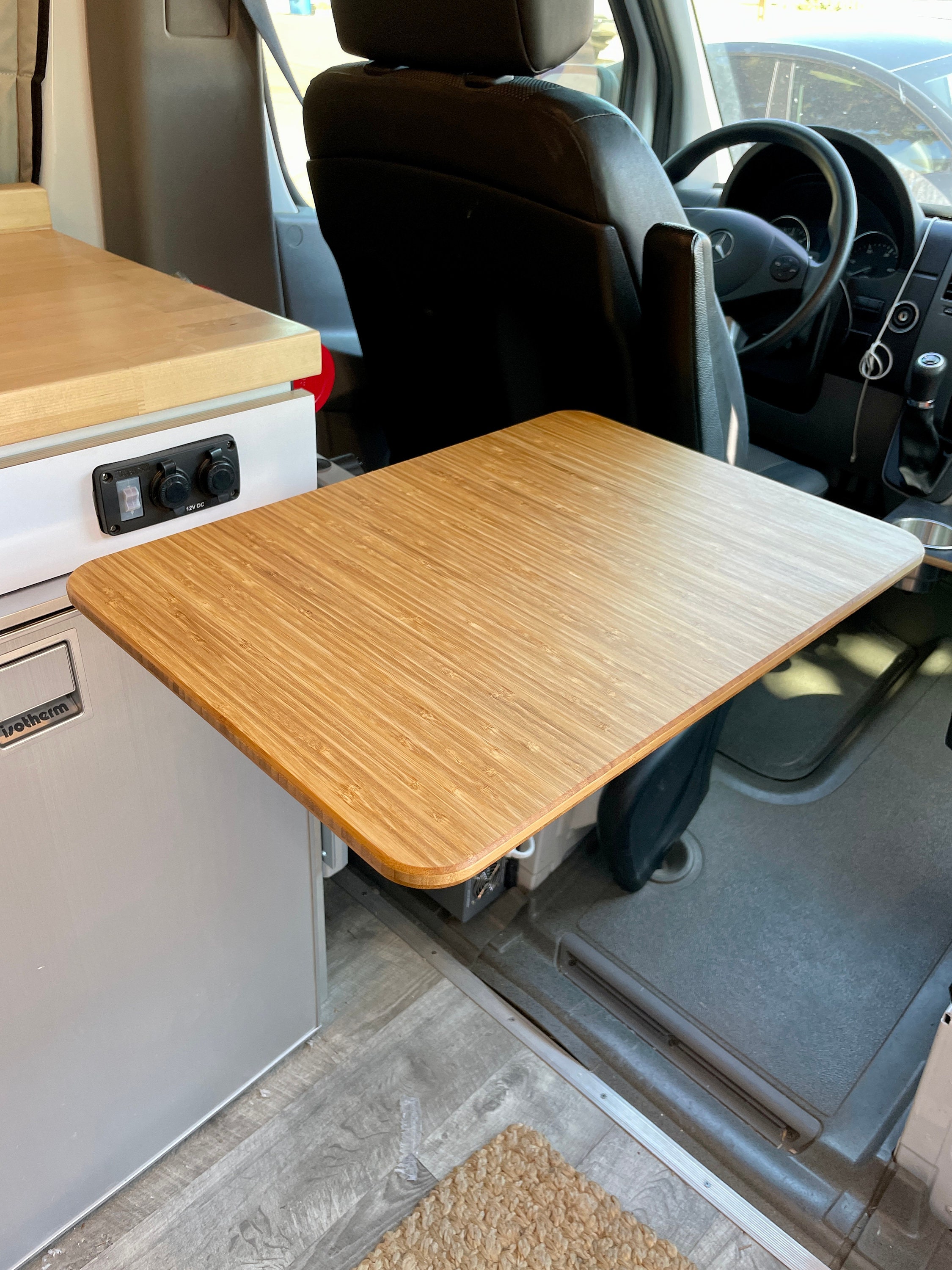This is a sharp, colored indoor photograph capturing the interior of a camping van or RV, taken during the daytime. The focal point is the front cabin, looking forward towards the driver's seat. The driver's seat is black with a Mercedes-Benz logo on the steering wheel in clear view. The armrest is pushed back, and an empty cup holder can be seen beside the seat.

Directly behind the driver's seat is a rectangular, oak-finish wooden table that appears to be suspended from an arm, with no visible legs. Adjacent to the table is a kitchen appliance—possibly a small refrigerator or dishwasher—featuring a pine wood cutting board on top. The appliance has a silver drawer beneath it with a couple of black buttons on a white background.

The photo shows the windshield and a parked vehicle visible through it. Other details include a wooden floor and a mat, which contribute to the cozy, habitable ambiance. The image provides a clear, detailed look into the front section of a thoughtfully arranged and functional camping van.